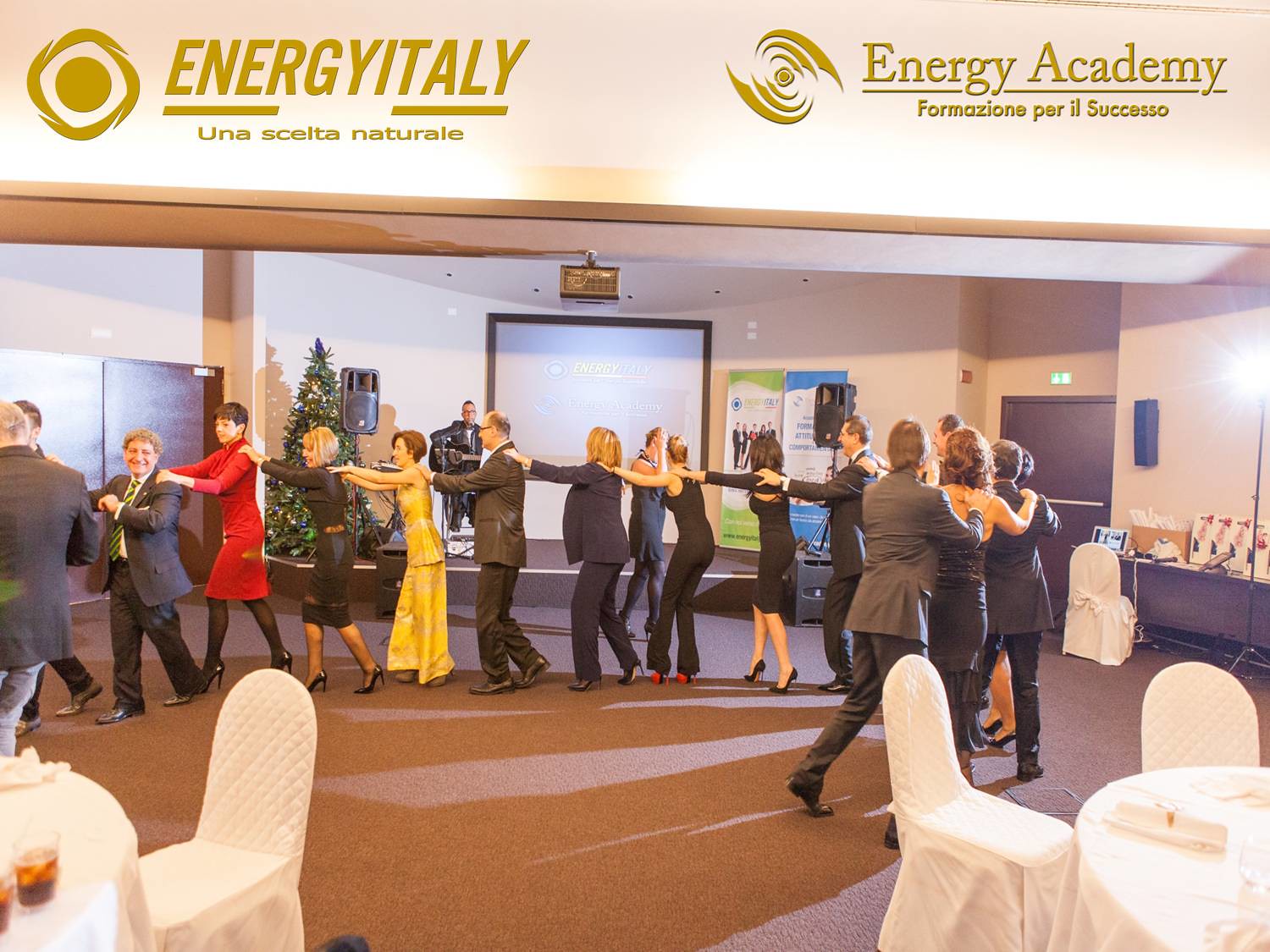This photograph, taken in an indoor convention center, captures a lively scene where approximately 15 to 20 men and women are participating in a conga line dance. The participants are dressed in a mix of suits and elegant dresses of varying colors, including red, yellow, and black. They dance with their hands on the shoulders of the person in front, forming an almost circular shape.

The background reveals more details about the setting: the walls are green, indicating a spacious hall used for events or gatherings. A stage is positioned in the front side of the hall, adorned with a musician who provides live music for the celebration, while a white projector screen displays visuals. Decorated tables and chairs, covered in white cloth, are spread throughout the room, contributing to the festive atmosphere. A decorated Christmas tree on the left side and a counter on the right with some materials on it further enhance the ambiance.

Above the scene, a banner reads "Energy Italy" in brown letters on a light beige background, accompanied by the "Energy Academy" logo. The event appears to be the "Energy Academy" convention, as indicated by the text at the top of the image. This celebratory gathering, centered around an academy promoting energy-related endeavors, brings a jovial and communal spirit to the attendees, evident from their synchronized dance and elegant attire.